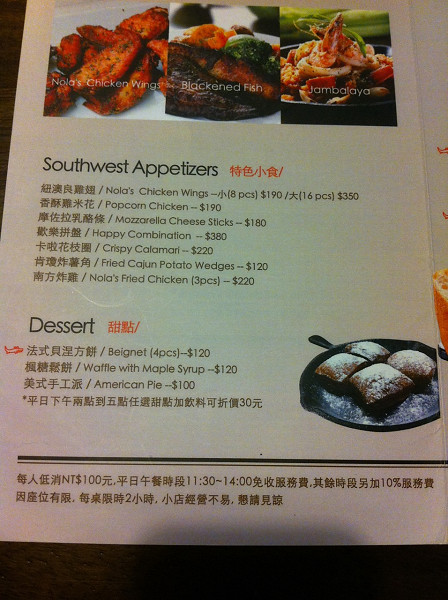The image showcases a bilingual menu featuring both Chinese and English text, presented on a table at a slight angle. The top third of the menu displays three enticing food images, each with descriptive text. On the left, an image with white text reads "Nola's Chicken Wings." The middle image features "Blackened Fish," and the image on the right showcases "Jambalaya." 

Beneath these images, bold lettering indicates the section of the menu dedicated to "Southwest Appetizers," written in black for the English text and red for the Chinese equivalent. This section lists seven delectable appetizers: Nola's Chicken Wings, Popcorn Chicken, Mozzarella Cheese Sticks, Happy Combination, Crispy Calamari, Fried Cajun Potato Wedges, and Nola's Fried Chicken, each accompanied by a price and corresponding Chinese translation.

Continuing down the page, the next section is titled "Dessert," offering three tempting choices: Beignet, Waffle with Maple Syrup, and Apple Pie. As with the appetizers, each dessert is listed with its price and an accompanying Chinese translation. The detailed organization and bilingual presentation make this menu both visually appealing and accessible to a diverse clientele.